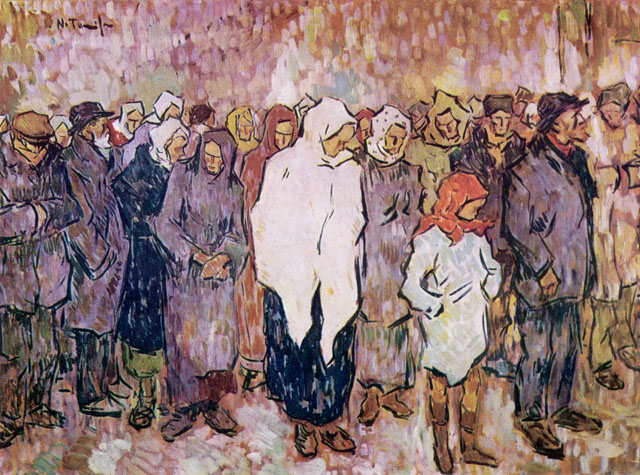This painting is a loosely impressionistic, slightly realistic depiction of a large crowd of somber-looking people, predominantly adults with one younger individual. The figures are positioned together, appearing to be waiting for something, possibly in cold or inclement weather, given their bundled-up attire. Many are wearing head coverings such as scarves or babushkas, while the rest sport hoods, suggesting an outdoor setting. The crowd, mostly clad in muted tones of white, purple, blue, and black, stands against a patchy, abstract background of pink, yellow, white, and brown hues, giving a sense of subdued mood. The scene's overall muted color palette and the downcast expressions of the figures contribute to the painting's melancholic and desolate atmosphere.